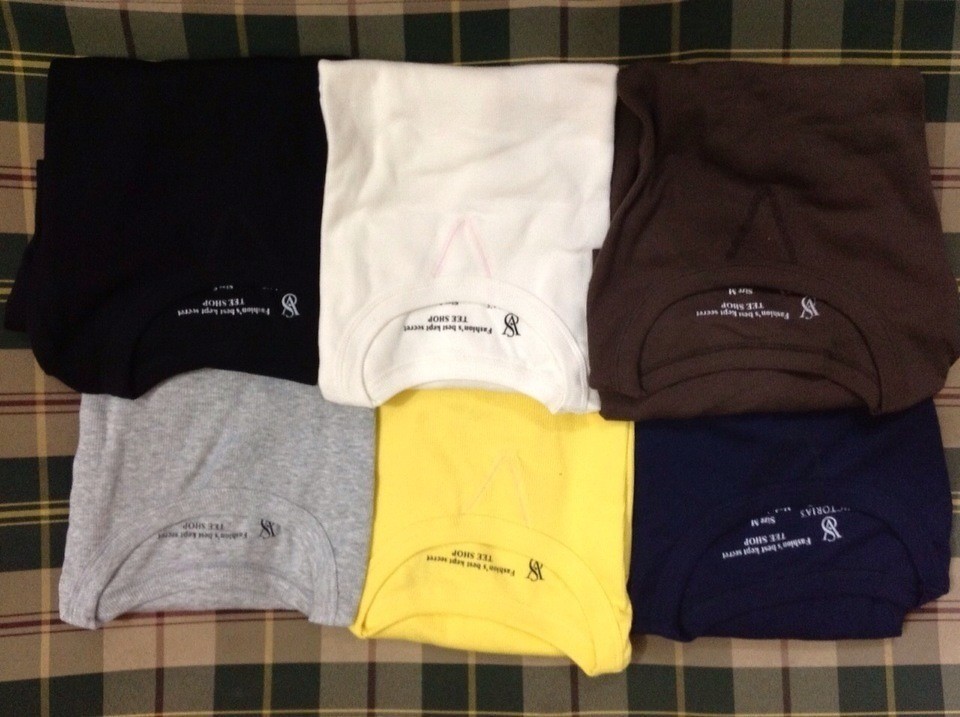Six Louis Vuitton t-shirts, all identical in style and size, are meticulously folded and arranged on a plaid surface featuring beige, black, and burgundy colors. The shirts are displayed in two neat rows of three, creating a visually pleasing layout. The top row consists of a black, a white, and a brown t-shirt, while the bottom row includes a gray, a yellow, and a dark blue t-shirt. Each shirt is folded in a way that obscures the sleeves, highlighting the logos on the inner collar: black writing on the white, gray, and yellow shirts, and white writing on the black, brown, and dark blue shirts. The plaid surface, possibly a couch cushion, enhances the presentation of these premium casual shirts.